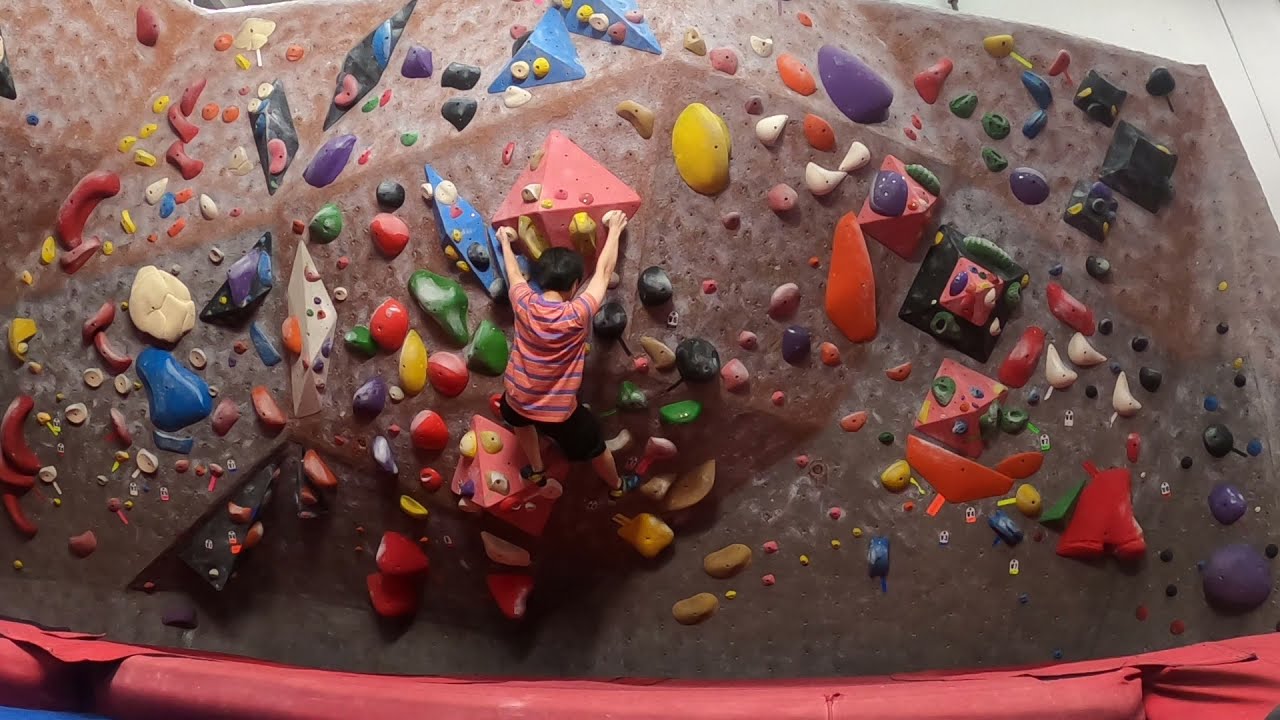This detailed image features a young boy climbing an indoor rock wall with a light brown background and a bright red bottom section. The entire wall is densely populated with a variety of colorful rock handles in shades of purple, orange, blue, yellow, white, green, and red. The boy, who has dark short hair, is dressed in an orange and purple striped shirt and black shorts. He is about halfway up the wall, gripping two small handles while his feet rest on one of the vibrant boulder holds. He appears to be looking down, and the wall includes sections that protrude outward, adding to the challenge. The bottom of the wall is padded, suggesting a safety cushion to protect climbers as they descend or fall. The boy is approximately three to four feet off the ground, demonstrating his adventurous climb on this vividly colored, multifaceted rock wall.